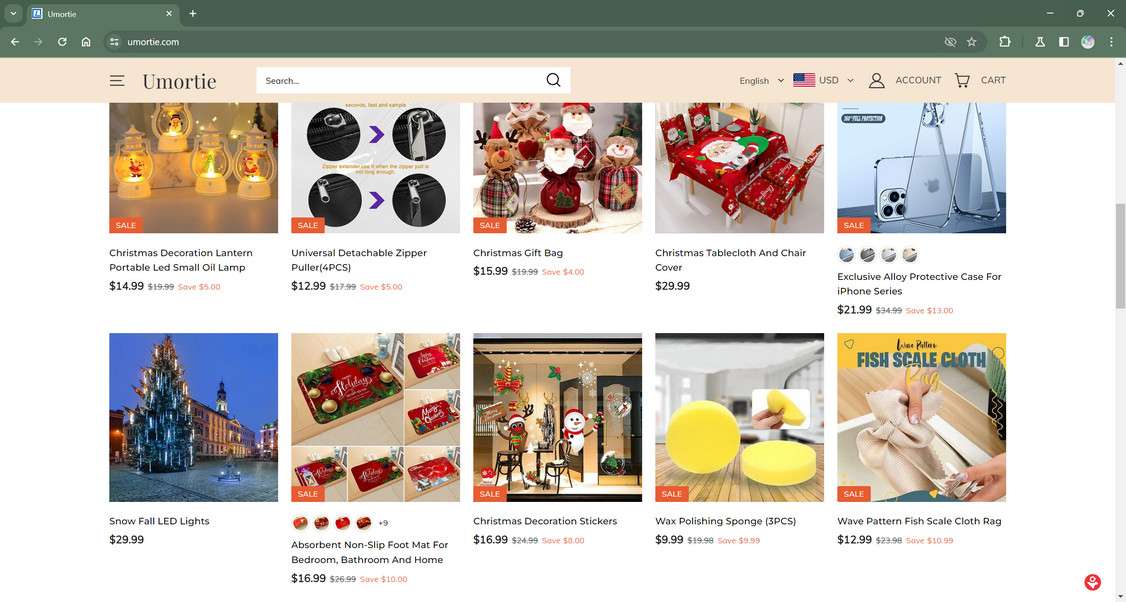The screenshot showcases the homepage of umortie.com as viewed on a web browser with a green header. The browser tab is labeled "Interesting." Below this, the website features a peach-colored header with a sleek layout. On the left side of the header, there is a hamburger menu icon, followed by the site’s logo centered in a search field. To the right, the header displays options for language selection (notably English), represented by an American flag with "USD" beside it. Additionally, there is an account icon and a shopping cart icon, the latter indicating items in the cart.

The main content area displays a grid of ten product thumbnails arranged in two rows of five. Each product is clearly represented with visuals and prices. Here are the detailed descriptions of the highlighted items:

1. **Christmas Decoration Lantern Portable Red Small Lamp** - Priced at $14.99, this product is visually represented as a small, red, portable lantern ideal for Christmas decorations. It includes a "Sale" badge.
   
2. **Universal Detachable Zipper Puller** - This item costs $12.99 and features a versatile and detachable zipper puller. It also has a "Sale" badge.

3. **Christmas Gift Bag** - Displayed with a price tag of $15.99, this product showcases beautifully decorated bags suitable for Christmas gifts, perfect for mantelpiece decorations. It includes a "Sale" badge.

4. **Christmas Tablecloth and Chair Covers** - Priced at $29.99, these items feature Santa-themed designs suitable for festive table settings. This product does not have a "Sale" badge.

5. **Exclusive Allied Protective Case from the iPhone Series** - Available for $21.99, this protective case appears durable with a clear design and metal rim, suitable for various iPhone models. It is marked with a "Sale" badge.

6. **Snowfall LED Lights** - These LED lights, depicted illuminating a large Christmas tree outside a significant government plaza, are priced at $29.99 and have a "Sale" badge.

7. **Assortment of Non-Slip Foot Mats** - These mats, suitable for the bedroom, bathroom, and home, announce phrases like "Merry Christmas" and "Happy Holidays." Priced at $16.99, this product includes a "Sale" badge.

8. **Christmas Decoration Stickers** - Priced at $16.99, these festive stickers include images of a reindeer, snowman, and other holiday figures displayed on a window. They carry a "Sale" badge.

9. **Wax Polishing Sponge, Three Pieces** - At $9.99, this set includes three yellow, wedge-shaped sponges, designed for polishing tasks. They are under the "Sale" category.

10. **Fish Scale Cloth, Wave Pattern Fish Scale Cloth Rag** - For $12.99, this product features cloth rags with a distinct fish scale pattern, suitable for various cleaning needs. It is also promoted with a "Sale" badge.

This detailed view provides a comprehensive glimpse into the festive offerings available on umortie.com, highlighting both functional and decorative items suited for the holiday season.